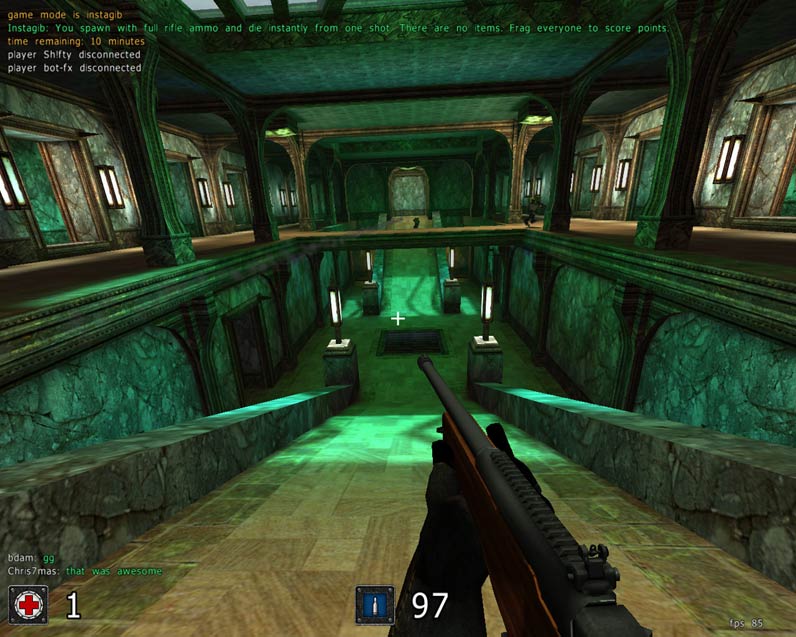The image depicts a first-person shooter video game interface set within a corridor characterized by a marine-ish green-blue and various shades of brown. The viewpoint is from a character holding a rifle, notably a black shotgun with a brown stock, gripped by a hand in a black glove. The player, who has an on-screen health indicator displaying a single life in the lower left corner, seems poised at the top of a beige and brownish-green slide or ramp. The slide, flanked by low walls on each side, leads down to a small block, atop which stands a white light pole. Upon reaching the bottom, the player encounters four pedestals with light fixtures and a central square, potentially a trap, drain, or tunnel entrance. The environment is structured with concrete walls and brown concrete columns, featuring a mix of dark and light brown tones, with marble-patterned design elements and numerous windows on the second floor, supported by many pillars. The rifle's bullet count, displaying 97, is visible above the character's hand. The overall setting hints at a vaguely subterranean or enclosed area, suggesting an intricate, multi-level game environment.